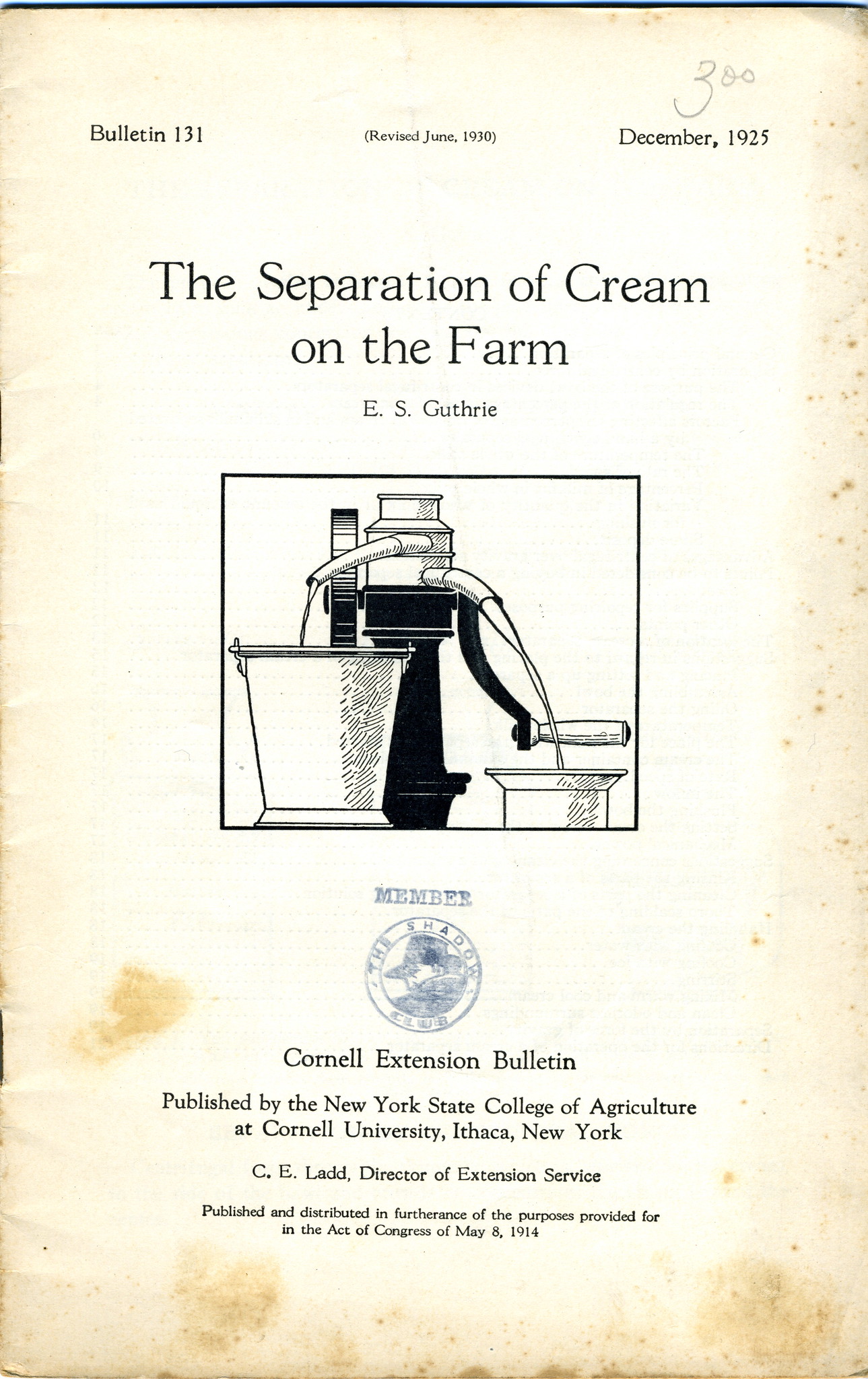This is a color photograph of a very old bulletin entitled "The Separation of Cream on the Farm" by E.S. Guthrie. The document is marked as Bulletin 131, with a revision date of June 1930 and an original publication date of December 1925. Centrally featured is a detailed drawing of a cream-separating device, which appears to funnel cream into two different buckets. Above the December 1925 date, a handwritten note in pencil lists a price of $3, suggesting it was likely purchased used. Below the illustration, the text reads "Cornell Extension Bulletin, published by the New York State College of Agriculture at Cornell University, Ithaca, New York, C.E. Ladd, Director of Extension Service. Published and distributed in accordance with the purposes provided for in the Act of Congress of May 8, 1914." The overall appearance of the bulletin suggests it is printed on very old paper, with all text in black font.